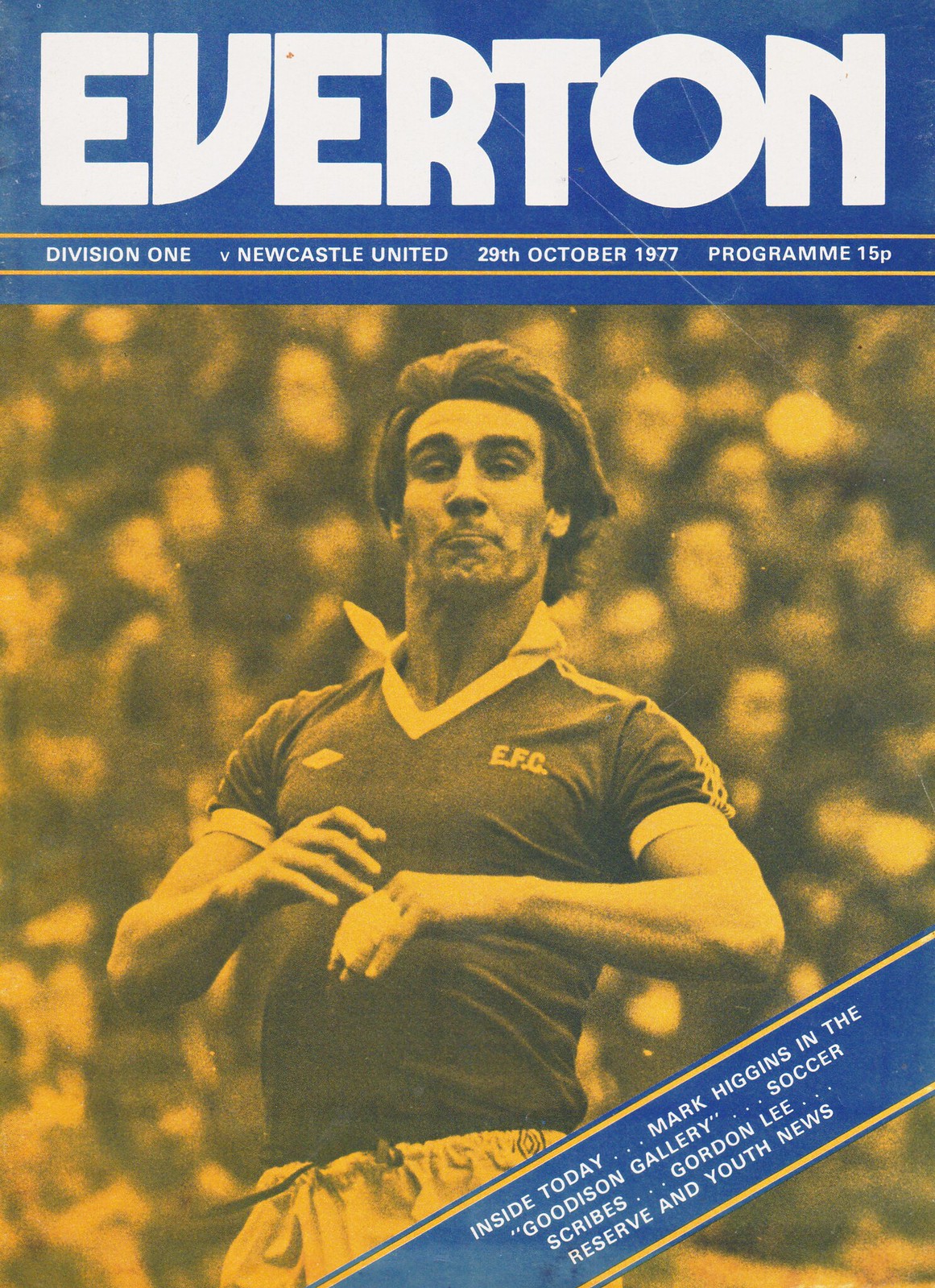The image is a vintage sports program cover from an Everton Football Club match against Newcastle United, dated 29th October 1977. The top of the cover features a blue, horizontal rectangle with the title "Everton" in large white capital letters. Directly below this, a smaller strip with gold borders details the subheading: "Division 1 vs. Newcastle United, 29 October 1977, Program 15 pence."

Central to the cover is a sepia-toned action photograph of a soccer player in mid-run, arms raised, and sporting a subtle smirk. The player, possibly around his late 20s with dark hair, is dressed in a jersey and shorts, with an emblem that looks like "EFC." In the background, spectators in the stands are faintly visible, adding to the vintage ambiance of the image.

At the bottom right of the cover, a diagonal banner in white font on a blue background with a gold border lists the contents of the program: "Inside Today: Mark Higgins and the Goodison Gallery, Soccer Scribes, Gordon Lee, Reserve and Youth News." This detailed and historically rich cover captures the essence of a bygone era in football program design.